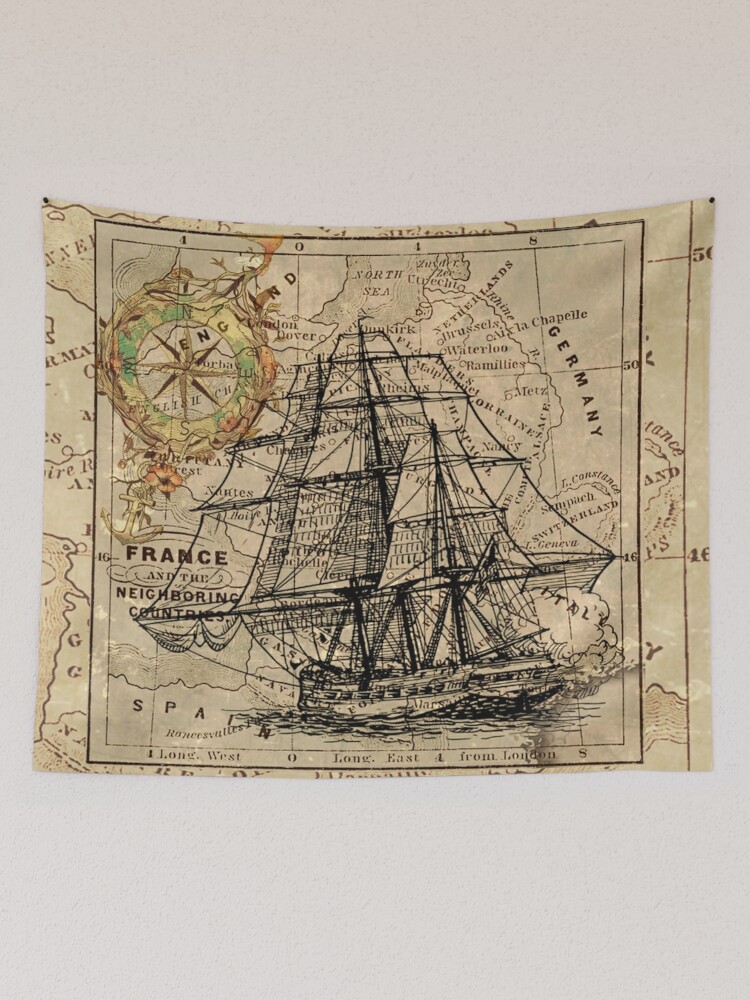The image depicts an antiquated, yellowed map set against a light gray background. The map features a detailed black and white ink drawing of a galleon-type sailing ship, likely from the 1400s or 1500s, with all sails billowing. The ship is illustrated on the waters, and though the scene does not show any crew, it includes windows along the ship's sides.

On the map, various European countries are labeled, such as Germany, France, Spain, Switzerland, and Italy. The North Sea is prominently marked, as well as Dover. There are horizontal latitude and longitude lines crisscrossing the map, with some difficult-to-discern writing accompanying these lines at both the top and bottom.

In the top left corner, there is a compass rose designed as an eight-pointed star, adorned with green and red, making it resemble leaves and flowers. The map appears to be pinned to a wall with black pins on the top edges. The labels also mention some directional coordinates like "Lake 10LS" and Long East/West from London, adding to the historical navigational feel.